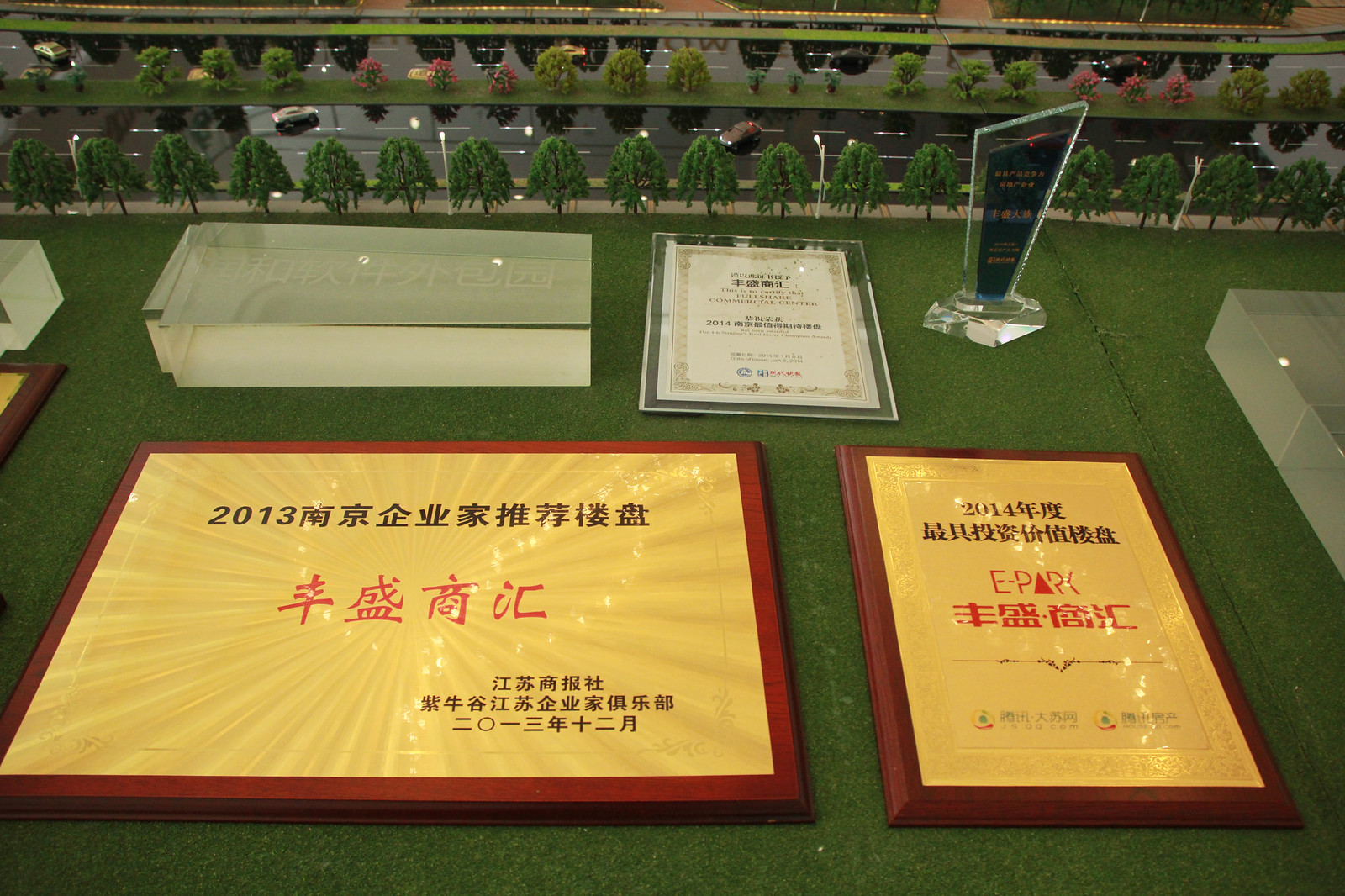The image depicts a detailed miniature setup resembling an urban planning model, complete with a black road marked with lines, tiny matchbox cars, and miniature trees on a green, possibly AstroTurf, surface. In the foreground, there are two large plaques, both with a yellow background, red characters, and a wooden base. The larger rectangular plaque on the left displays the year 2013, while the taller, thinner plaque on the right is marked with the year 2014 and the word "e-park." Both plaques are written in Asian characters, likely Japanese. Behind the plaques, there is a box, and various trophies are visible, including a clear, almost triangular glass trophy and another white, milky glass trophy. The backdrop features abundant greenery with numerous trees. The overall impression is that of an award ceremony or presentation, potentially related to urban planning, given the detailed miniature environment and multiple awards present.